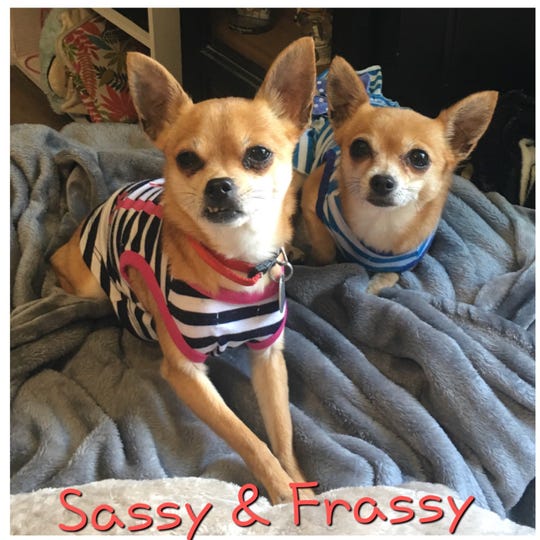The image captures a cozy indoor scene, likely set in the living room of someone's house. Central to the photo are two small chihuahuas lying on a spread-out blue blanket that covers the majority of the bottom half of the frame. The chihuahuas are positioned in the center of the image, exuding a sense of comfort and slight menace. The dog on the left, identified as "Sassy," is adorned in a black, pink, and white striped shirt, while the one on the right, known as "Frassy," sports a blue and white striped shirt. Both dogs have brown fur with lighter faces. Placed directly beneath them, the text "Sassy & Frassy" in pink letters with a black outline prominently labels the pair. Behind the dogs, shelves holding various items occupy the upper portion of the image, suggesting a domestic setting. The plush gray velvet blanket and a few scattered pillows add to the relaxed and homely atmosphere.